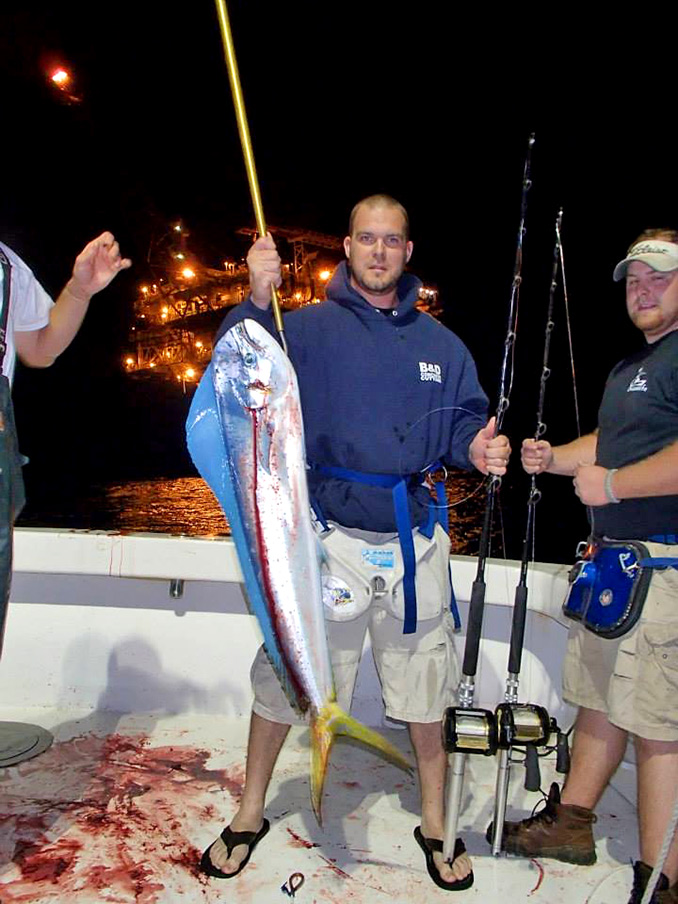At nighttime on a white boat, three men are pictured showcasing their fishing triumph. The central figure, clad in a navy blue hoodie emblazoned with the letters "BND" in white, and off-white khaki shorts, proudly holds a massive fish. This fish, nearly three-quarters the size of the man, boasts a silver-white body, blue fins, and yellow tail fins, with blood dripping down from it and splattered across the boat's deck. The man also holds a fishing pole in one hand and wears black flip-flops and a strap around his waist. To his right stands another man in a black T-shirt, beige shorts, brown work boots, and a beige visor, possibly marked with "Titleist," and equipped with fishing tools around his waist. This man is also holding a fishing pole. On the far left, barely visible, is a third individual whose presence is indicated by an arm clad in a white T-shirt and an apron, hinting at their involvement. The scene is set against a backdrop of a dark sky and distant lights, possibly from another boat on the water, emphasizing the nighttime fishing adventure.